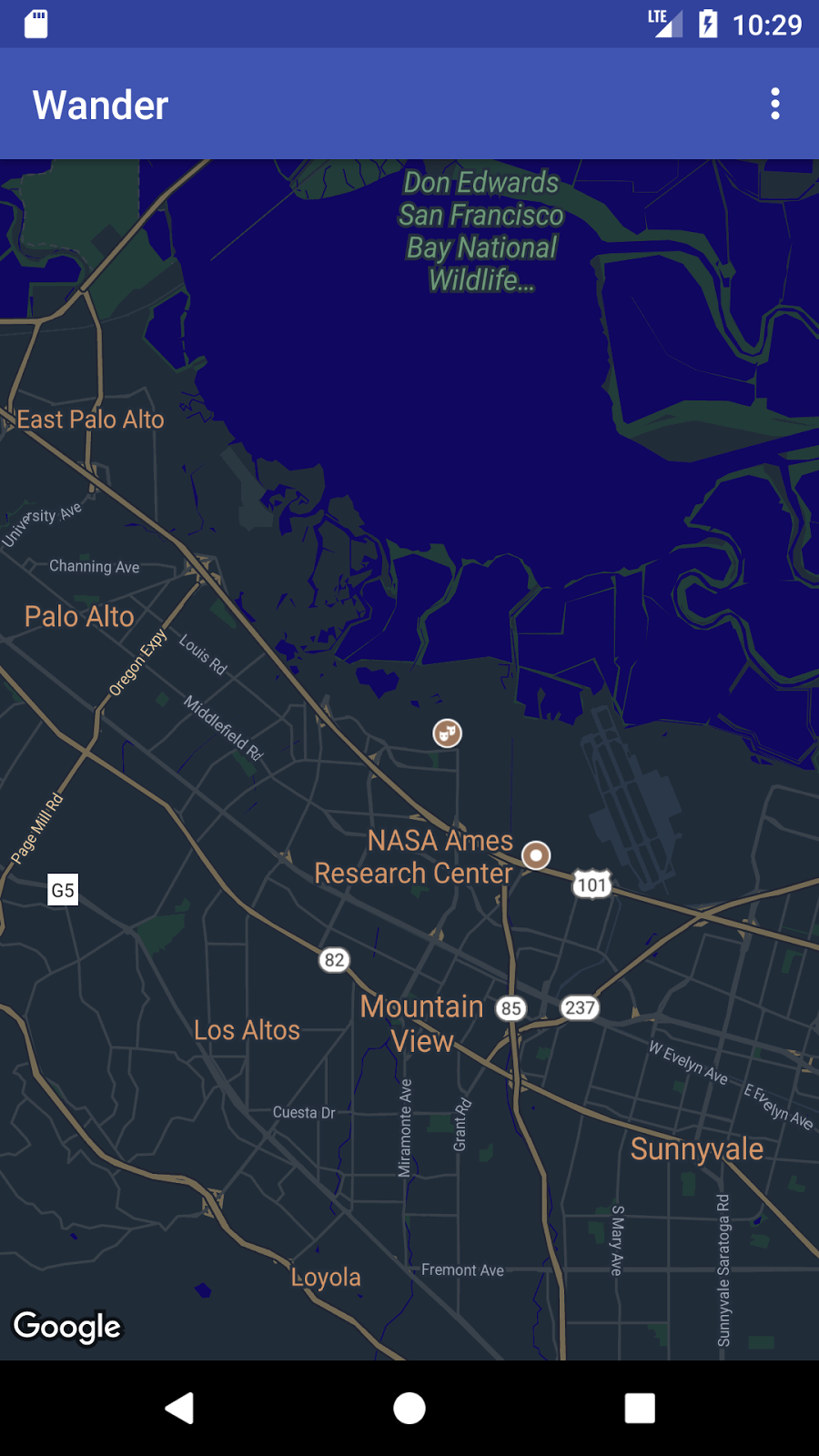The image appears to be a screenshot taken from a cell phone displaying a Google Maps interface. The top portion of the screenshot includes a blue bar, with the upper left corner showing a small icon resembling a memory card. In the upper right corner, indicators show a full LTE signal, a fully charged battery, and the current time as 10:29. Just below this, a lighter blue banner stretches across the top, featuring the word "WANDER" in bold white letters on the left and a clickable three-dot menu on the right.

The main section of the screenshot displays the map view, highlighting various locations in the San Francisco Bay Area. Prominently labeled on the map is "Don Edwards San Francisco Bay National Wildlife Refuge." Below this, the names of several nearby areas are visible, including "East Palo Alto," "Palo Alto," "NASA Ames Research Center," "Mountain View," "Los Altos," "Sunnyvale," and "Loyola." 

In the bottom left corner of the image, the word "Google" is displayed in bold white letters. The bottom of the screenshot features a black navigation bar with three icons: a left-pointing triangle on the left, a circle in the center, and a square on the right.